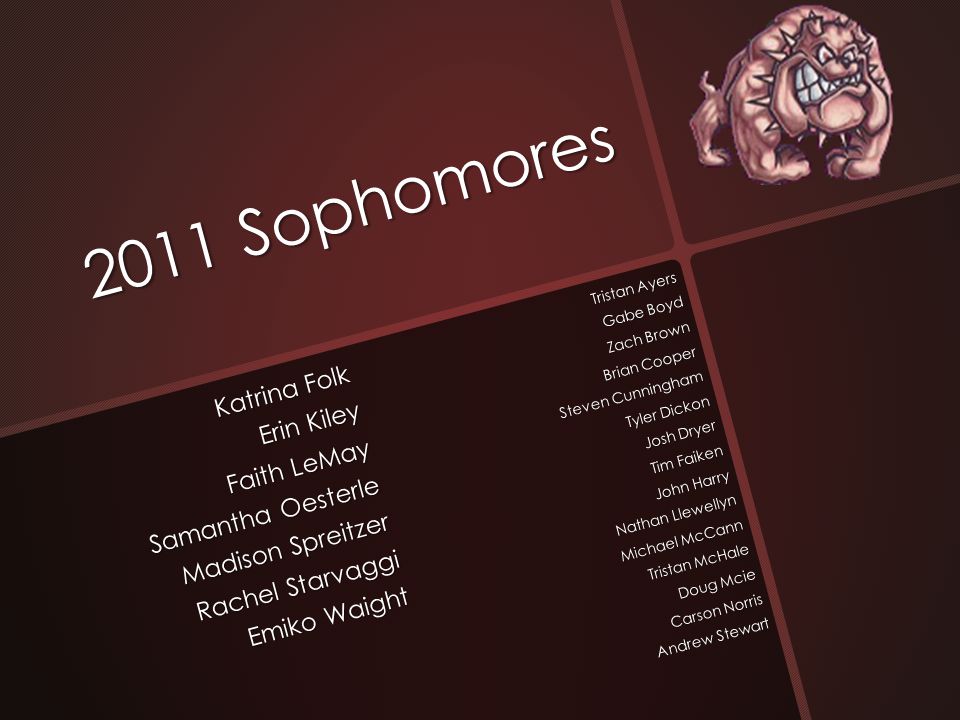The image is a horizontally aligned, maroon-themed graphic divided into four sections by two perpendicular diagonal red lines. The top left quadrant, which transitions from brighter maroon to darker shades, features the title "2011 Sophomores" in large, white, Comic Sans-like font that follows the diagonal line. Below this section is a darker maroon box listing two columns of students' names in small white text, right-aligned: Katrina Folk, Erin Kiley, Faith LeMay, Samantha Oesterle, Madison Spreitzer, Rachel Starvaghi, Emiko Waite, Tristan Ayers, Gabe Boyd, Zach Brown, Brian Cooper, Stephen Cunningham, Tyler Dicken, Josh Dreyer, Tim Fiken, Nathan Llewellyn, Tristan McHale, Michael McCann, Doug McKee, Carson Norris, and Andrew Stewart. The upper right segment displays a cartoonish, fierce-looking pinkish bulldog with a spiked collar, muscular physique, and bared teeth. This section's background is a dark maroon, nearly black in the corner. The lower right section consists solely of a gradient from dark to lighter maroon with no other elements. This graphic appears to be a school-related item such as a card or a PowerPoint slide.